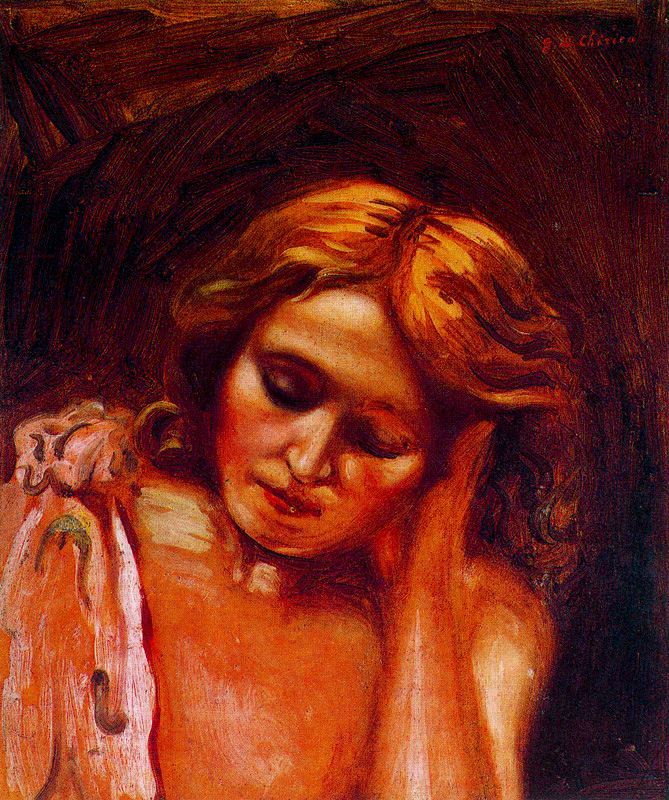This is an oil painting titled by Giorgio De Chirico from 1933, featuring a woman with a surrealistically rendered appearance, possibly painted in low light at sunset. The background is a dark palette, predominantly black with rich tones of orange and reddish-brown hues. The centerpiece, the woman, is portrayed with an orange-tinted medium skin tone. Her hair is reddish-brown, wavy, and shoulder-length, parted in the middle.

The woman is mostly nude, with a piece of salmon-colored fabric draped over her right shoulder. This cloth seems to be a dress or shirt, ambiguously covering her chest. Her eyes are closed, and her expression is serene, accentuated by the soft detailing of her face, which includes medium brown eyebrows, a hint of brown eyeshadow, and pink to red lips. She is gently cupping the left side of her face with her left hand while her head and eyes tilt downward. The painting is a masterful exercise in contrasts and muted orange tones, contributing to its distinct surrealistic style.